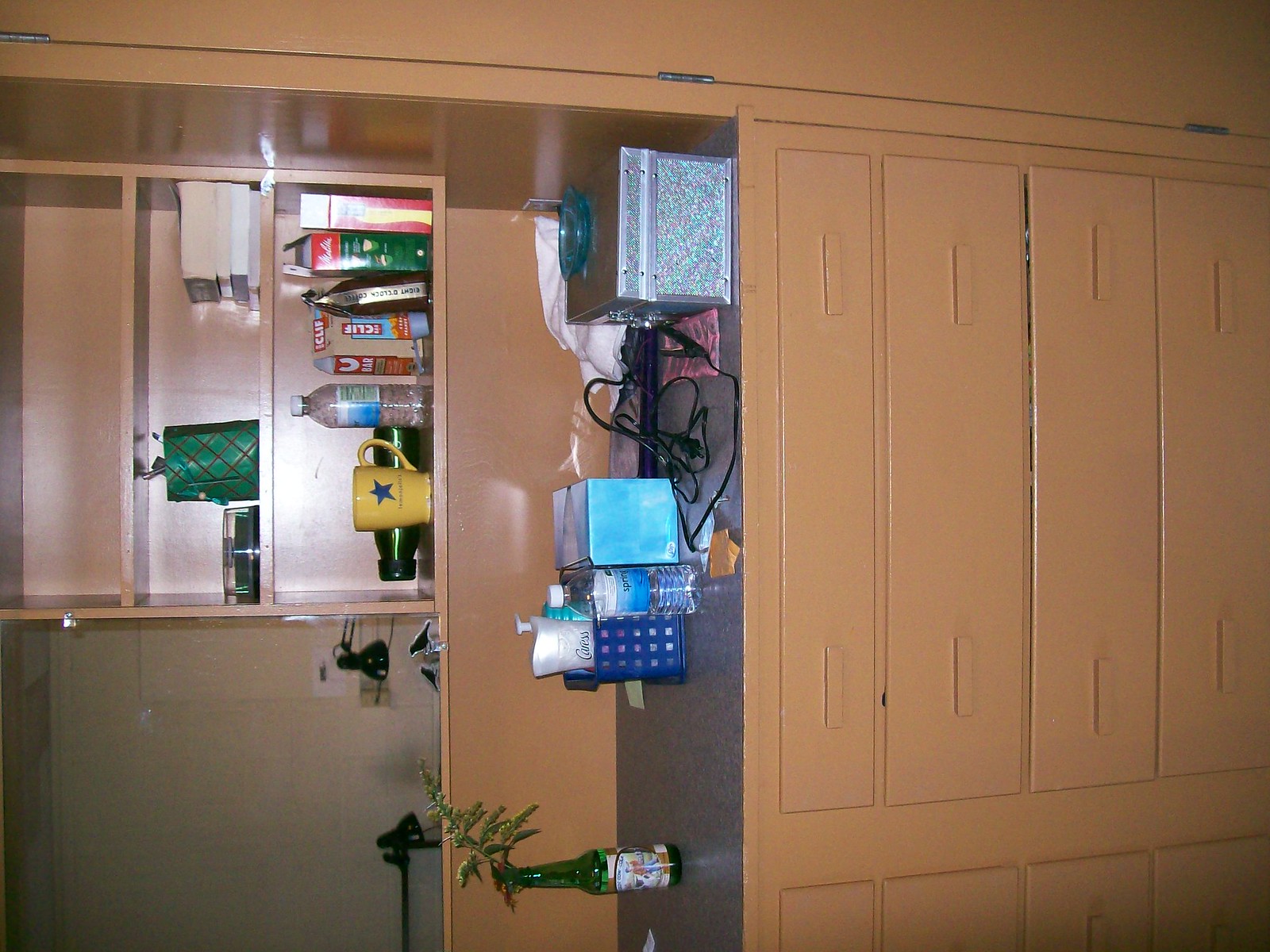This image depicts a built-in dresser situated in a bedroom. The dresser, predominantly brown, is turned sideways in the image and would need a one-step rotation to the right to be properly oriented. The dresser features four drawers at the bottom, topped by a laminate countertop. Above the countertop is a space that leads to three shelves positioned to the right, and on the left, there appears to be a mirror.

From left to right, the first item on the shelf is a green glass bottle filled with flowers. Beside it, there is a blue basket containing a stick of Caress deodorant and a bottle of lotion behind it. A box of tissues and a water bottle are situated next to the basket. Further to the right, a laptop lies with its black cord visible. At the far right end of the shelf, there is an iridescent jewelry box topped with an aquamarine glass tray, which likely serves as a ring holder.

On the bottom shelf, there is a yellow coffee cup decorated with a blue star, placed in front of a green water bottle lying on its side. Next to the coffee cup, there is a plastic water bottle, a box of Clif Bars, and three other unidentified boxes.

The middle shelf holds four books, a gift bag, and some type of plastic container. Reflected in the mirror, two black lamps can be seen, adding to the room's ambiance.